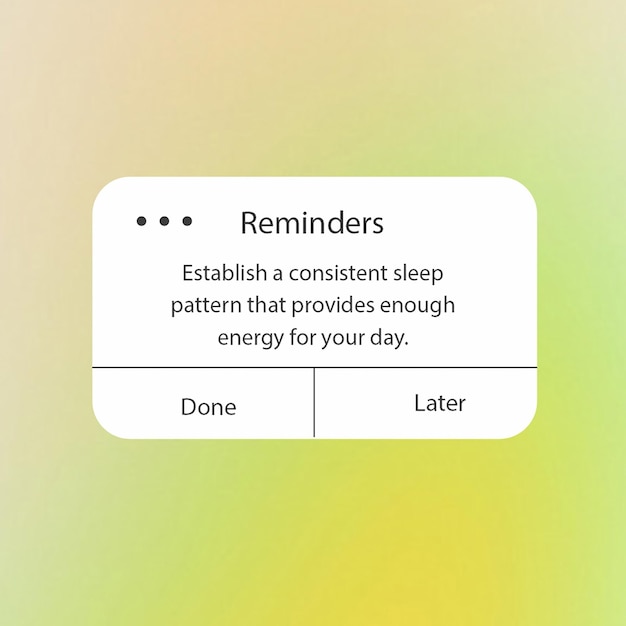The image features a gradient-colored box transitioning from peach to light green, ending in a yellowish-orange hue. Within the box, there is a prominent white square that contains a reminder message written in black text. The reminder emphasizes the importance of establishing a consistent sleep pattern to maintain adequate energy levels for the day. Below the message, there are three ellipsis dots, followed by a long horizontal line. At the bottom of the white square, the options "Done" and "Later" are presented for interaction. The overall design is simplistic and focuses on the reminder and its associated actions.